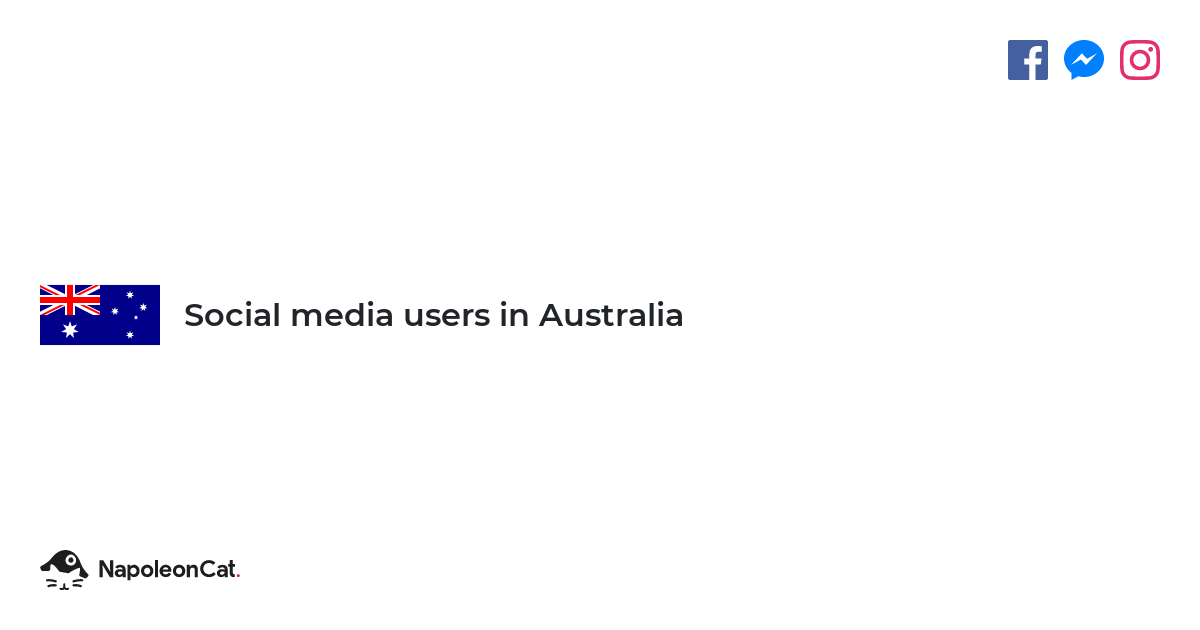The image features a blank white backdrop. In the top right corner, there is a red square with a white interior. It is outlined in white and has a white button with a small pink dot above it, indicating an icon for Instagram. To the left is a blue speech bubble icon with a white lightning bolt running horizontally across it, representing Facebook Messenger. Next, there is a dark blue square with a lowercase white "f" slightly to the right of the center, symbolizing Facebook.

Moving down about halfway and to the far left, the Australian flag is depicted. The flag is blue with a red X and a red cross superimposed on top. It features a six-pointed star, a seven-pointed star, four smaller stars, and one tiny dot. Beside the flag, in black text, it reads "Social Media Users in Australia," with "Australia" and "Social" capitalized.

In the bottom left corner, there is the outline of a black hat with a small black dot inside a white circle, resting on top. Below the hat, black whiskers emerge, indicating the outline of a cat's face with a small mouth at the center. Beneath this, in bold black text, it reads "Napoleon Cat" with a red period at the end.